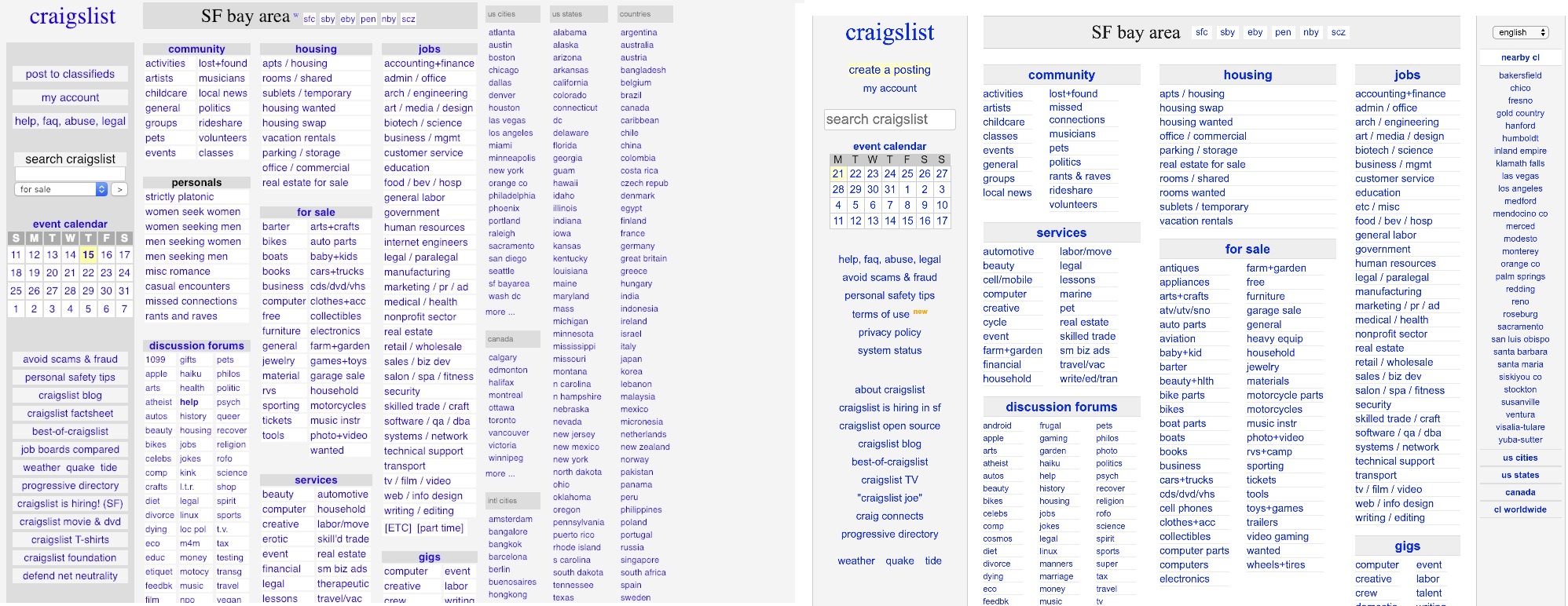This image features two screenshots from the Craigslist website, specifically displaying the Craigslist homepage for the Santa Fe Bay Area. 

The left screenshot showcases the site's vertical navigation menu, which includes numerous sections such as "post to classifieds," "my account," "help," "FAQ," "abuse," "legal," "search Craigslist," "event calendar," "avoid scams and fraud," "personal safety tips," "Craigslist blog," "Craigslist fact sheet," "best of Craigslist," "job boards compared," "weather," "quake," "tide," "progressive directory," "Craigslist is hiring," "SF," "Craigslist movie and DVD," "Craigslist t-shirts," "Craigslist foundation," and "defend net neutrality." Below the navigation menu, different categories are listed, which include "community," "personals," "discussion forums," "housing," "for sale," "services," "jobs," and "gigs."

The right screenshot mirrors the left but focuses on displaying a list of different cities, states, and countries where Craigslist is accessible. In addition, a new section listed under the categories is highlighted in orange text labeled "terms of use," indicating recent updates.

Both screenshots collectively provide a detailed overview of the Craigslist homepage, elucidating its extensive navigation options and the wide geographic availability of its services.